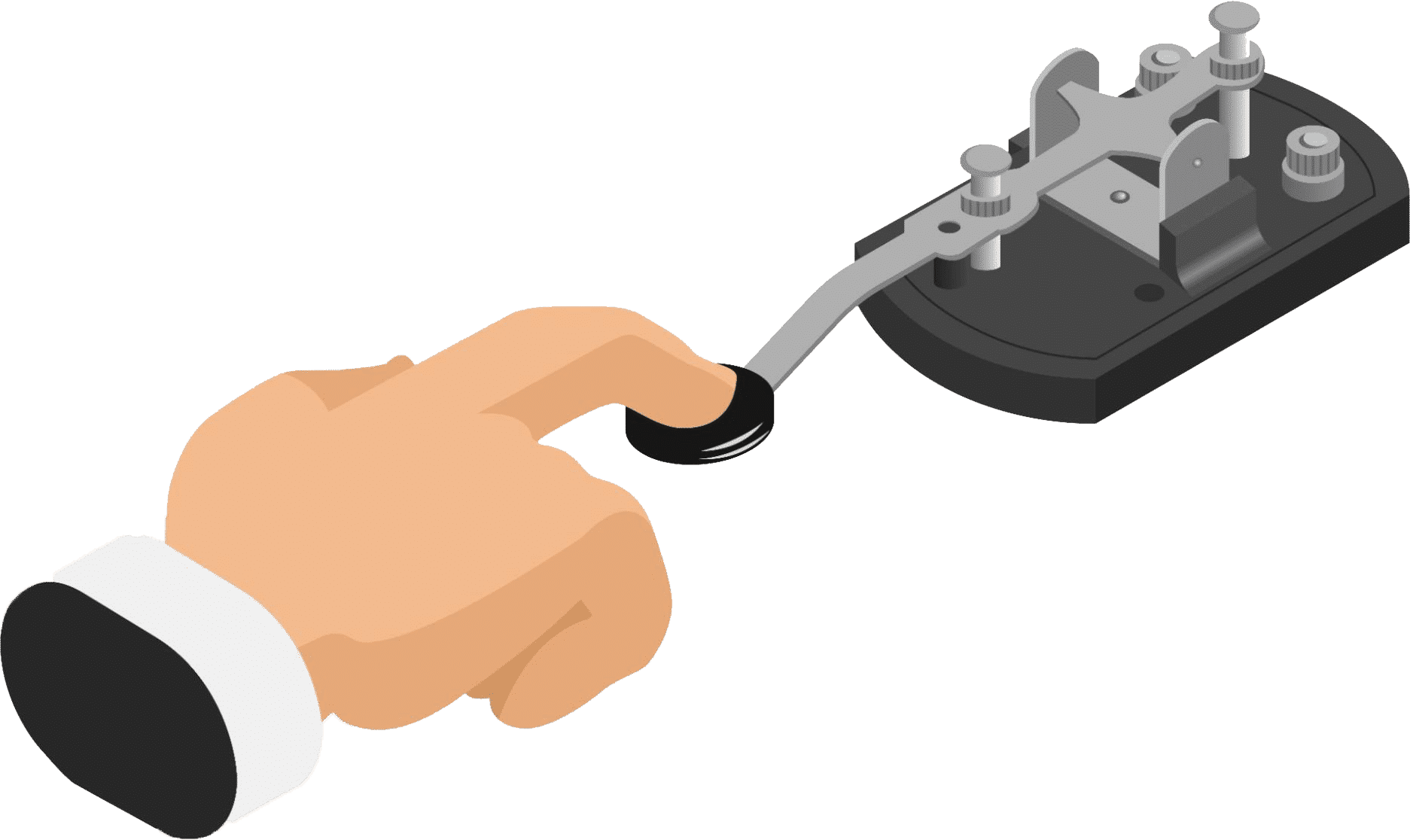This is a digitally illustrated cartoon depicting a hand operating a telegraph machine. The hand, shown in the bottom left of the image, has a white collar on the wrist and extends to press the button on the telegraph with its middle finger. The telegraph machine features a black end attached to a gray bar with screws, extending back to the main component. The main body of the telegraph is black and silver. The white background helps to draw attention to the detailed, mechanical parts of the telegraph and the deliberate action of the hand, emphasizing the historical process of sending a telegraph message in Morse code.